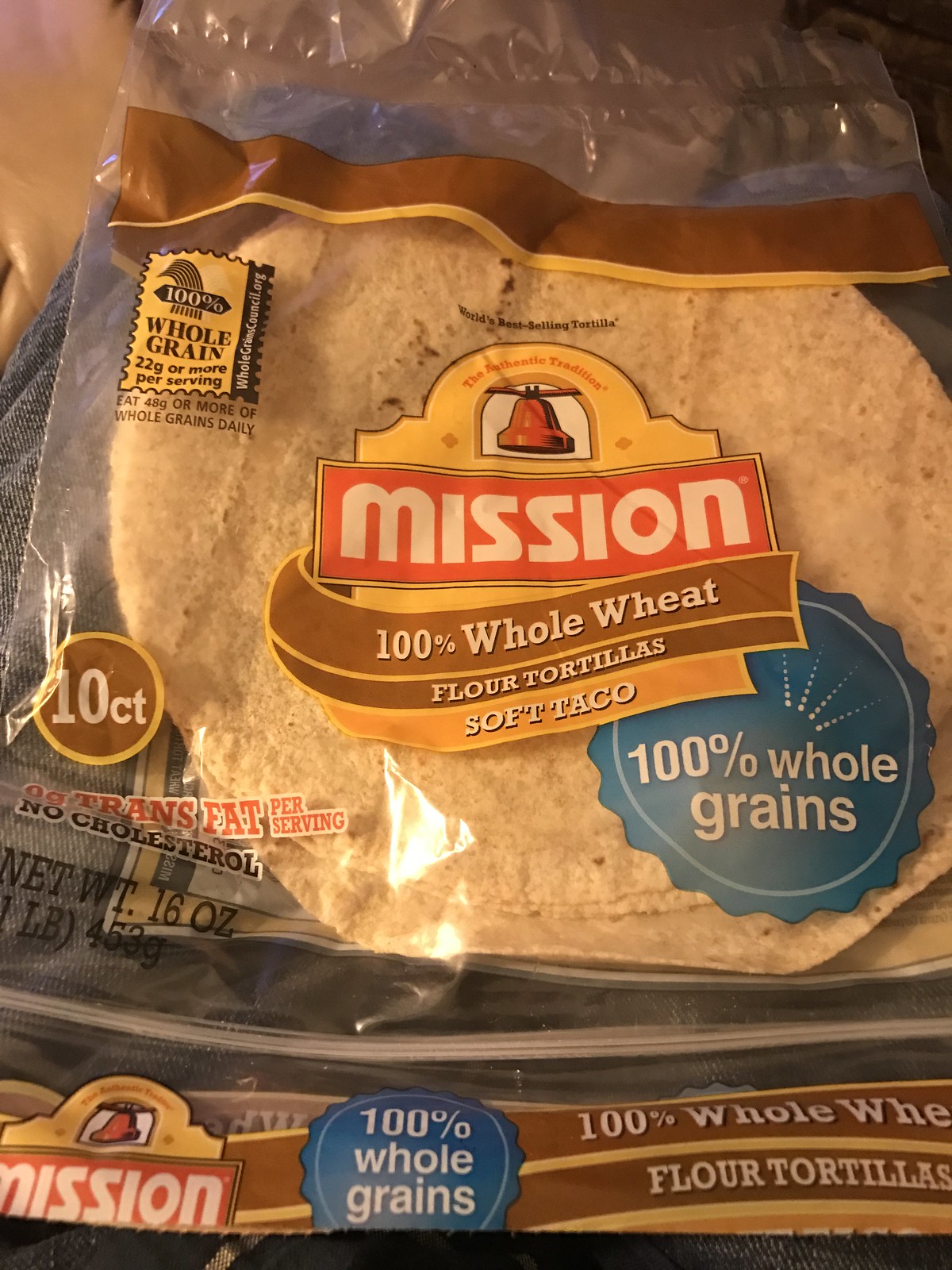This image features a clear plastic bag containing Mission's 100% Whole Wheat Flour Tortillas. The brand's distinctive design includes the iconic bell logo in the center with "The Authentic Tradition" above it, and "Mission" prominently displayed. Below the brand name, the bag indicates "100% Whole Wheat Flour Tortillas Soft Tacos" and highlights that these tortillas are made with 100% whole grains. To the right, a circular icon displays "100% Whole Grain," while on the left, it notes "10 count," denoting the quantity of tortillas, which is clearly visible through the see-through packaging. The net weight is listed as 16 ounces (453 grams), approximately one pound. The upper left corner of the bag features an icon stating "World’s Best Selling Tortilla" along with nutritional details, mentioning that each tortilla provides 22 grams or more of whole grains per serving and advising to consume 48 grams or more of whole grains daily.